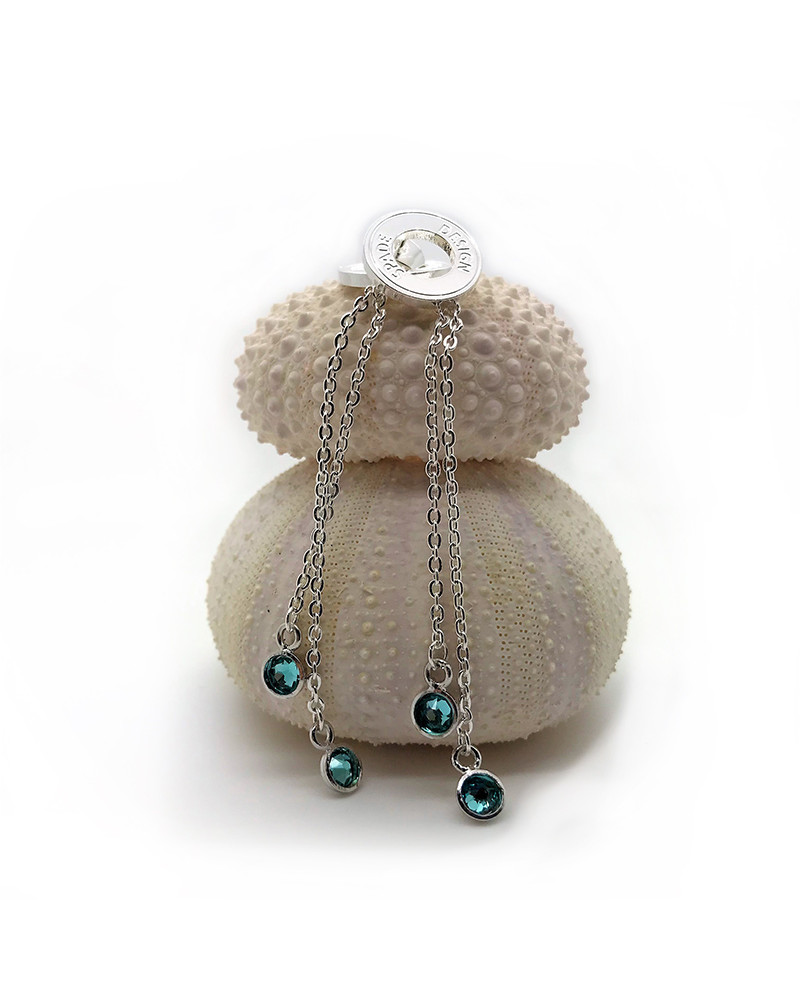The photograph features two stacked cushions in a whitish cream color. The top cushion has a spiky texture, while the bottom one displays a dotted pattern. Resting atop these cushions is a round silver medallion with unintelligible engraved text. Attached to the medallion are silver chains adorned with circular blue turquoise gemstones. The background of the image is white, providing a clean and minimalist contrast that highlights the details of the cushions and the jewelry.